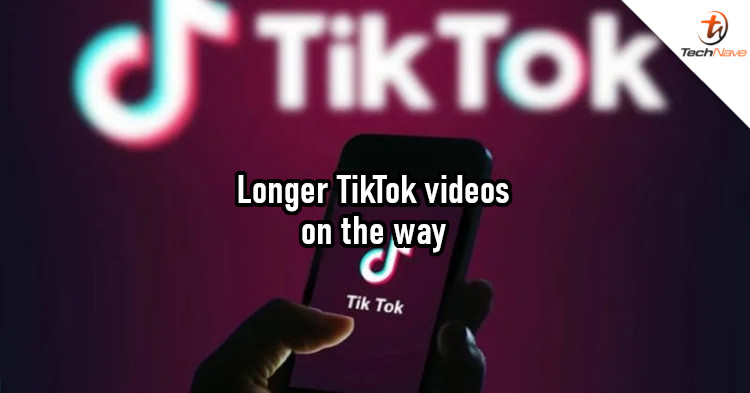The image is a vibrant TikTok advertisement with a richly detailed background. The backdrop features a deep eggplant purple hue, particularly pronounced on the left and right edges, while the center transitions to a brighter magenta tone. At the top center, the iconic TikTok emblem and the word "TikTok" appear in white, though the text is slightly blurry. 

In the upper-right corner, there is a distinctive white area containing an outlined circle with orange and black borders. Inside the circle, a "T" is scribbled. Just below this, the text "Tech Knave" is displayed, with "Tech" in black and "Knave" in orange.

Dominating the bottom center of the image is a prominent left hand holding a smartphone. The thumb, ring finger, middle finger, and pinky are distinctively visible. The phone's design is sleek, with a rectangular shape and curved corners. Its outer edge is black, and the screen displays a purple background featuring the white TikTok emblem and the word "TikTok." Adding to the advertisement's message, white text with black trim is superimposed over the phone's screen, proclaiming, "Longer TikTok videos on the way."